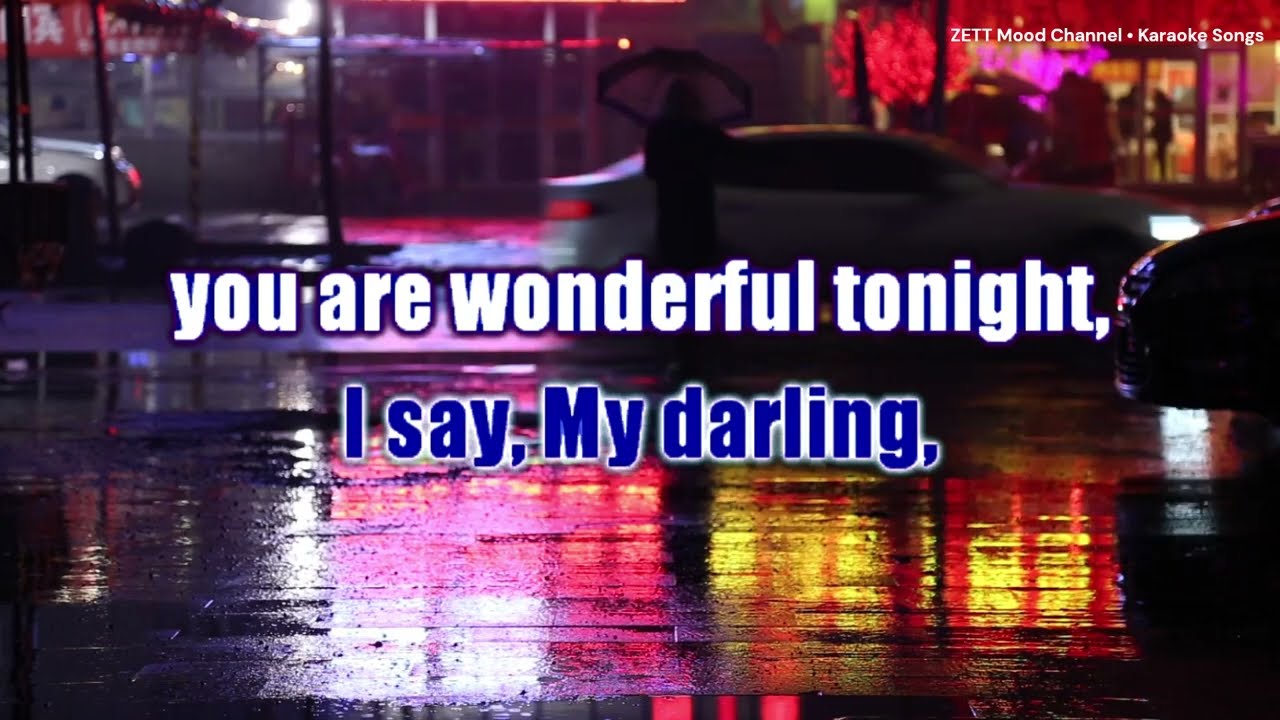In this vibrant, nighttime city street scene, rain-slicked pavement reflects a kaleidoscope of colorful city lights in hues of red, pink, yellow, orange, purple, and blue. At the foreground, a silhouetted figure holding an umbrella walks towards a vehicle, adding a solitary, introspective mood to the image. Several cars are parked or passing by, with at least a white car in the middle, a black car to the right, and another white car parked on the left. The bustling activity is softened by the rain, creating puddles that capture the light and enhance the scene’s vividness. In the center of the image, large white Impact font letters bordered in royal blue spell out, "You are wonderful tonight," followed by a line below in navy blue Impact font with capitals, "I say my darling." The text hints at song lyrics, possibly for a karaoke rendition, adding a sense of romance and nostalgia. In the upper right corner, small white text reads "ZET Mood Channel • Karaoke Songs," indicating this image might be from a video thumbnail or a channel promoting karaoke content. The overall scene is one of urban beauty and lyrical emotion, captured in a moment of reflective solitude.